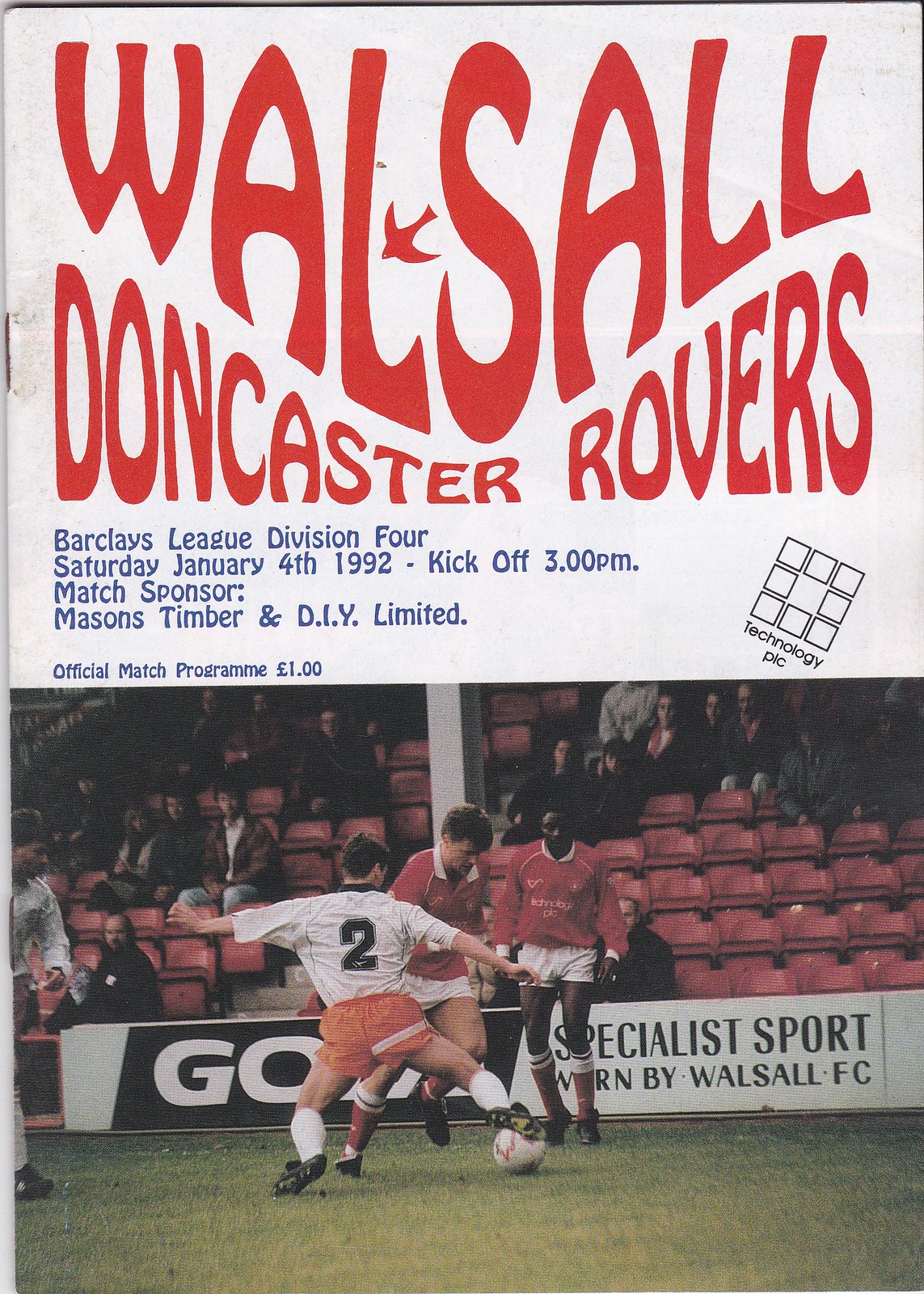This is an image of an official match program booklet from January 4, 1992. The program is divided into two sections. The top section has a white background with red lettering that reads "Walsall Doncaster Rovers" in a distinct font that fades from small to large. Below that, in blue ink, it states "Barclays League Division 4," followed by "Saturday, January 4, 1992, kickoff 3 PM." The next lines include the match sponsor "Mason's Timber and DYI Limited" and the price, "Official match program, One Pound." There is also a Technology PLC logo present. The lower section features a vintage photograph of an actual soccer match on green turf. In the image, two soccer players in red long-sleeve jerseys with white collars and white shorts are competing against an opposing player dressed in a white jersey with black numbers and orange shorts. Additional players and a backdrop of seats filled with spectators are visible, with a partially legible sign in the stands reading "Go [unreadable] Specialist Sport."